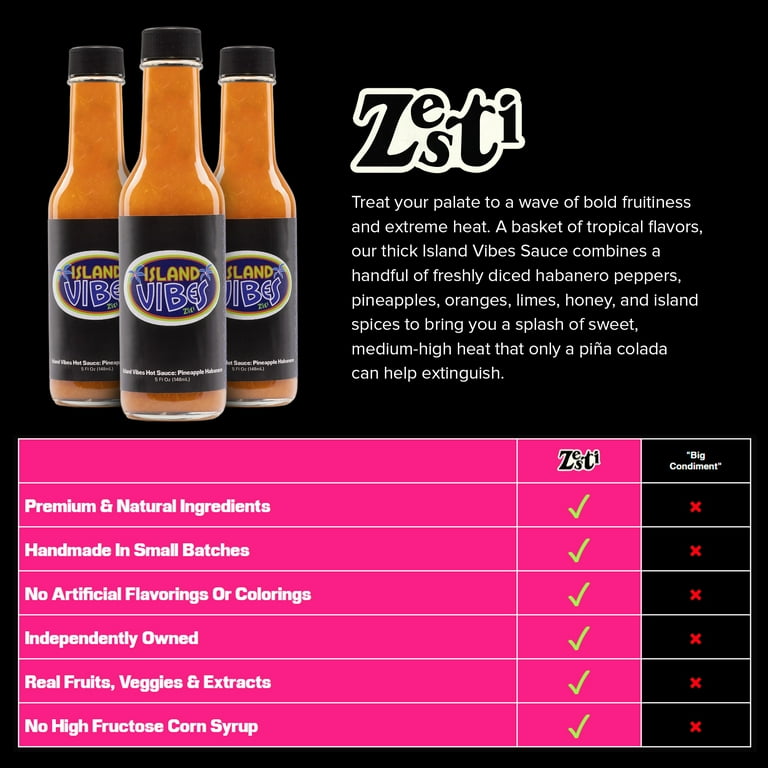The image features a large, square format with a solid black background. In the upper left corner, there are three identical glass bottles with black caps and black labels containing a brown liquid. The labels display the text "Island Vibes," where "Island" is in light brown and "Vibes" is in blue outlined in white. In the upper right corner, the text "Zesty" appears, with the letters creatively arranged so that the "E" is on top of the "S," all against a white backdrop in black letters. Beneath this logo, left-aligned text describes the product: "Treat your palate to a wave of bold fruitiness and extreme heat. A basket of tropical flavors, our Thick Island Vibes sauce combines a handful of freshly diced habanero peppers, pineapples, oranges, limes, honey, and island spices to bring you a splash of sweet medium-high heat that only a piña colada can help extinguish." At the bottom of the image, a horizontally aligned, rectangular table with six to seven rows and three columns showcases various criteria. The first column is unlabeled. The second column, labeled "Zesty," features multiple yellow check marks indicating positive attributes, while the third column, labeled "Big Condiment," has red X's, highlighting a lack of those same qualities. Some of the criteria include premium and natural ingredients, handmade in small batches, no artificial flavorings or colorings, independently owned, real fruits, veggies, and extracts, and no high fructose corn syrup.